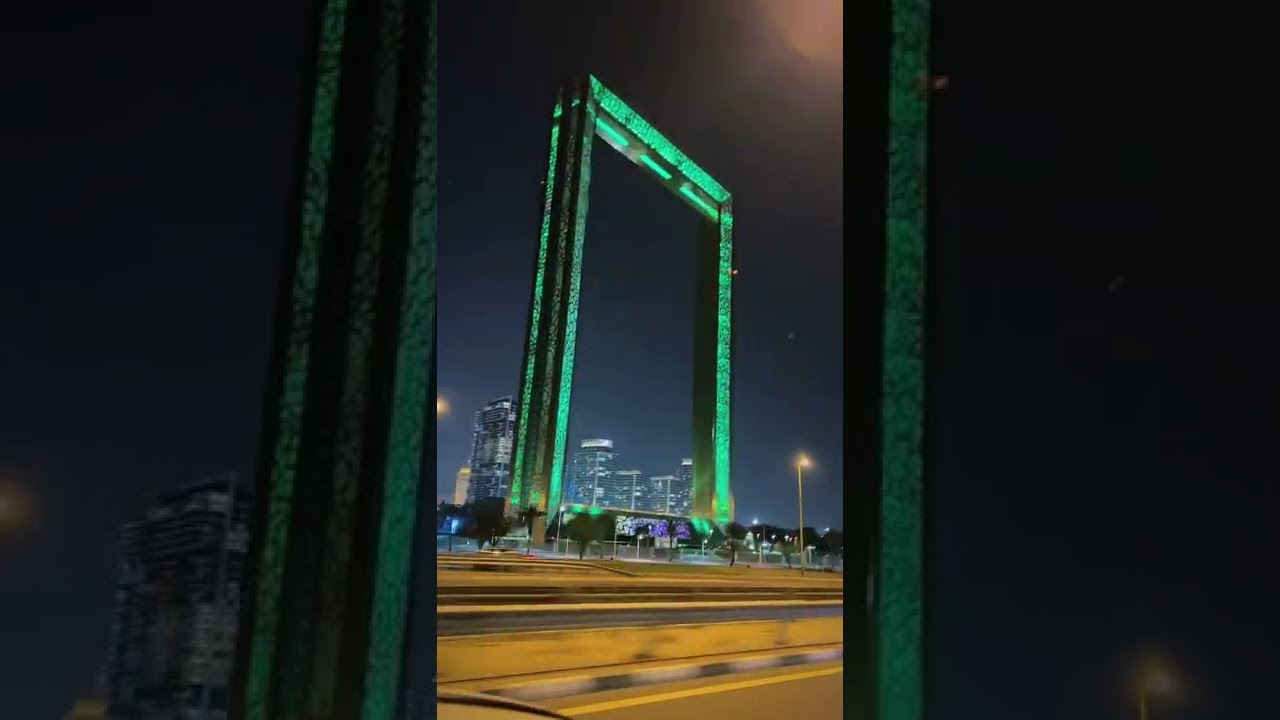This image features a wide rectangular composition centered on a tall, rectangular photograph of a modernistic arch within a cityscape. Flanking this central photograph on either side are darker, close-up portions of the same arch, creating a dramatic contrast. The bottom section of the image showcases a road adorned with yellow barriers, slanting upwards diagonally, leading to a small fence that marks the beginning area of the arch itself.

The arch, a prominent element in the picture, appears to be crafted from a black material intricately illuminated by bright green neon stripes that emphasize its architectural lines. This striking structure extends vertically from nearly the bottom to the top of the frame, with two straight pillars on either side and a flat top, forming a monolithic silhouette.

Enveloped in the nighttime setting, the dark sky and the scattered gleam of city lights and windows enhance the arch's luminous presence. The entire scene exudes an urban nightscape, with colors predominantly comprising black, various shades of green, yellow, gray, and additional hues like brown, blue, and purple provided by the distant city lights. The contrast between the arch's vibrant neon glow and the subdued background elements creates a visually captivating ambiance, reflecting the interplay between modern architecture and the surrounding urban environment.